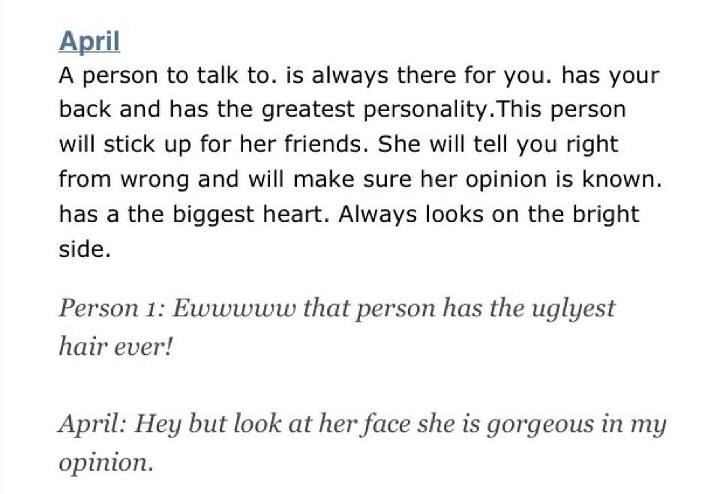On a plain white background, a print piece titled "April" appears at the top left in blue, underlined. Below, in black text, it describes a person who is always there for you, has your back, and possesses the greatest personality. This individual will stand up for her friends, offer moral guidance, make her opinions known, has the biggest heart, and always maintains a positive outlook. The text features poor grammar and punctuation, with many sentences lacking capitalization at the beginning. Further down, in blue italics, are text exchanges between "Person One" and "April." Person One exclaims, "Eww! That person has the ugliest hair ever!" To which April responds, "Hey, but look at her face. She is gorgeous, in my opinion." The piece captures a brief dialogue alongside a character description, highlighting contrasting perspectives on beauty.